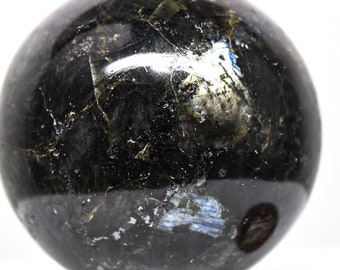The image depicts a glossy black bowling ball with intricate patterns featuring white streaks and splotches, and subtle hints of light blue. The ball, albeit cropped at the top and bottom edges, showcases a detailed white splosh in the center that extends to the left. Additionally, there's a light blue splash near what appears to be a finger hole at the bottom right corner. The glossy surface, marked by gray highlights, reflects light and the table it rests on, emphasizing the ball's smooth finish. Though the image is of low resolution, the intricate design gives the ball a marble-like appearance with hints of other colors, possibly olive or gold, adding to its allure.